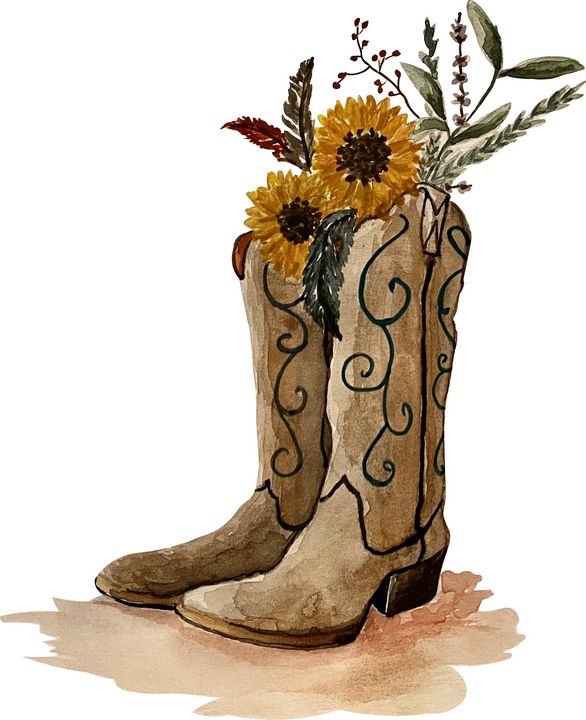The image is a detailed painting with a completely white background. At its center, there's a pair of brown cowboy boots, possibly painted with watercolor, featuring intricate black patterns running vertically up their long legs. The boots are characterized by a line running down the middle and bear pointy toes and dark brown heels, giving them a distinct cowboy style. The base of the boots contrasts with a smudgy, reddish-brown splotch, as if splashed with paint. Emerging from the top of the boots is a vibrant floral arrangement. Prominently, there are two sunflowers with black centers and yellow petals, surrounded by an assortment of additional foliage, including green and red leaves, twigs, and branches. Some stems with small berries are interspersed, making the boots appear repurposed as rustic, creative planters.